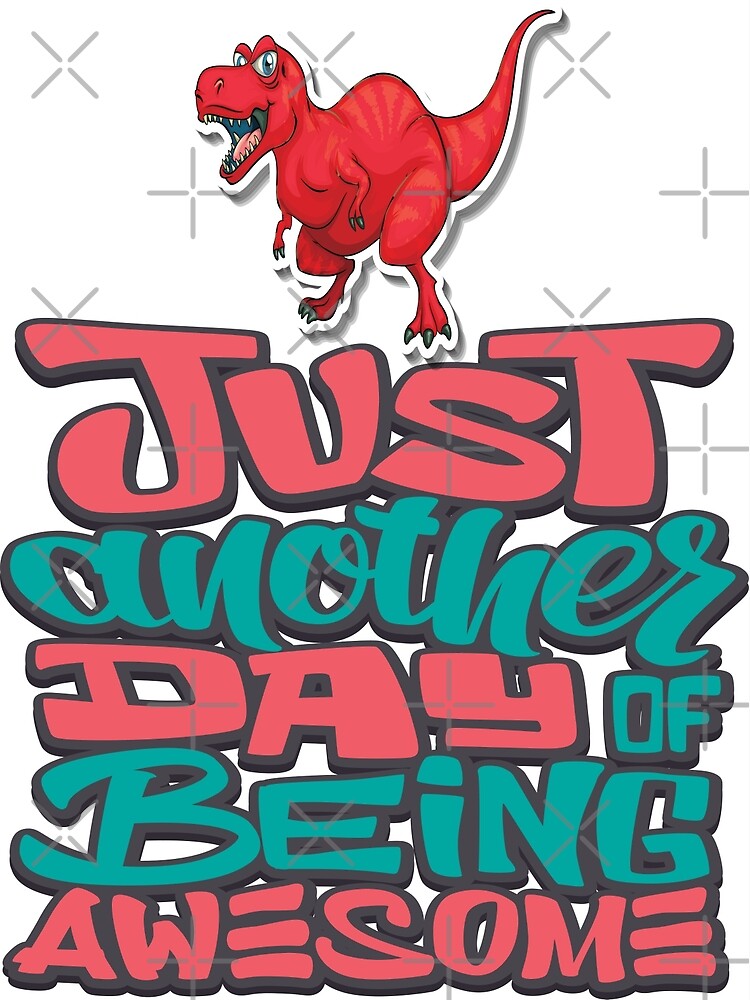This is a cartoon artwork featuring a red Tyrannosaurus rex at the top. The T-Rex, with its mouth open displaying numerous sharp teeth, has angry-looking white and blue eyes, gray claws, and a raised tail. Its body is primarily red with slightly lighter, orangish-red stripes. The dinosaur stands atop a graffiti-style text rendered in alternating colors by line: red and greenish blue. The text reads "just another day of being awesome." The background is a blank white, and the image is covered with small, faint Xs and crosses as watermarks that do not obscure the main illustration. This vibrant, full-body, non-photorealistic depiction of the T-Rex and text combination makes it suitable for merchandise such as t-shirts or stickers.